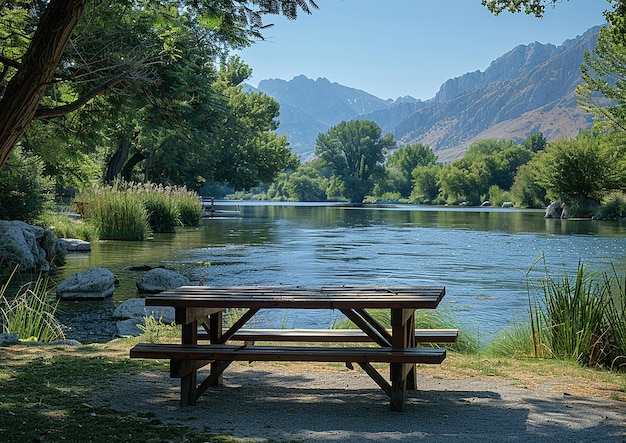This photograph captures a serene outdoor scene by a large, green lake, surrounded by lush trees and high, desert-style mountains, with a clear blue sky overhead. In the foreground, there's a dirt area where a wooden picnic table faces the lake, inviting one to sit and enjoy the tranquil view. The lake’s surface is mixed with areas of glass-like stillness and gentle ripples, with tall grass and large stones visible both in and around the water. Flanking the lake, tall, verdant trees add to the peaceful ambiance, while the backdrop showcases towering, earthy mountains. Cattails and various lake plants add to the natural beauty of the scene, making it a picturesque spot for relaxation and reflection.